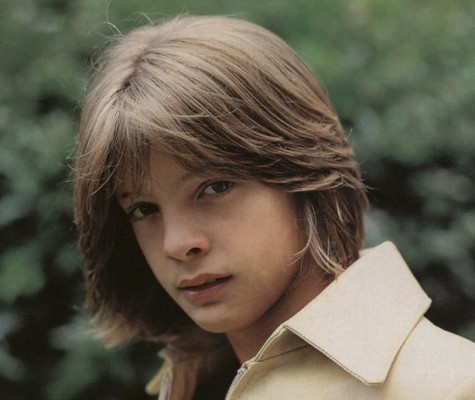This is a detailed portrait of a youthful Luis Miguel, likely taken in the 1970s. Standing outdoors, his figure is mostly oriented towards the bottom left corner of the image, but his head is slightly turned to face the viewer directly. His gaze, characterized by his brown eyes, adds a compelling focal point. Sporting thick, shaggy brown hair that cascades to intersect with his collar, it is brushed back on the sides while also falling over his forehead and covering his ears.

He is dressed in a tan, collared shirt that appears to be of a thicker material, maintaining a structured form that doesn't easily collapse. A lightly colored coat with visible zippers on both sides adds an extra layer to his outfit, though the shirt beneath remains obscured.

The background suggests an outdoor setting, dominated by blurred green vegetation, possibly trees or bushes. This blurred greenery heightens the focus on Luis Miguel. The lighting, seemingly from above, highlights the top part of his hair, accentuating the parting. His youthful appearance, paired with the natural backdrop, encapsulates a moment frozen in time, framed by nature's tranquility.